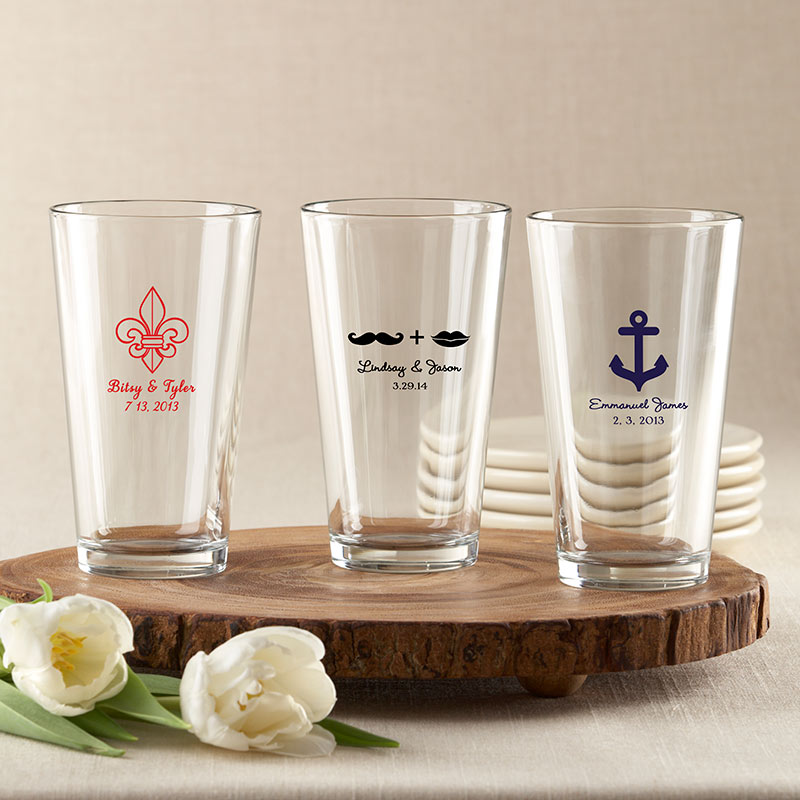The image showcases three tall glasses, each with distinctive designs and inscriptions, resting on a round piece of natural wood. The background features an off-white or cream-colored fabric with a subtle texture, resembling the appearance of a wall and table, respectively. 

To the right of the glasses, five small white round plates are neatly stacked. The glasses sit on a sealed wooden base, which has four half-circle pegs serving as feet. On the left side of the scene, white flowers, resembling tulips, and some leaves add a touch of nature to the arrangement.

From left to right, the glasses all appear similar in size and shape. The left glass displays a red Fleur de Lis symbol with the text "Betty and Tyler, 7-13-2013." The middle glass features a black mustache and lips, separated by a plus sign, along with the text "Lindsey and Jason, 3-29-14." The right glass is adorned with a navy blue anchor and the text "Emmanuel James, 2-3-2013."